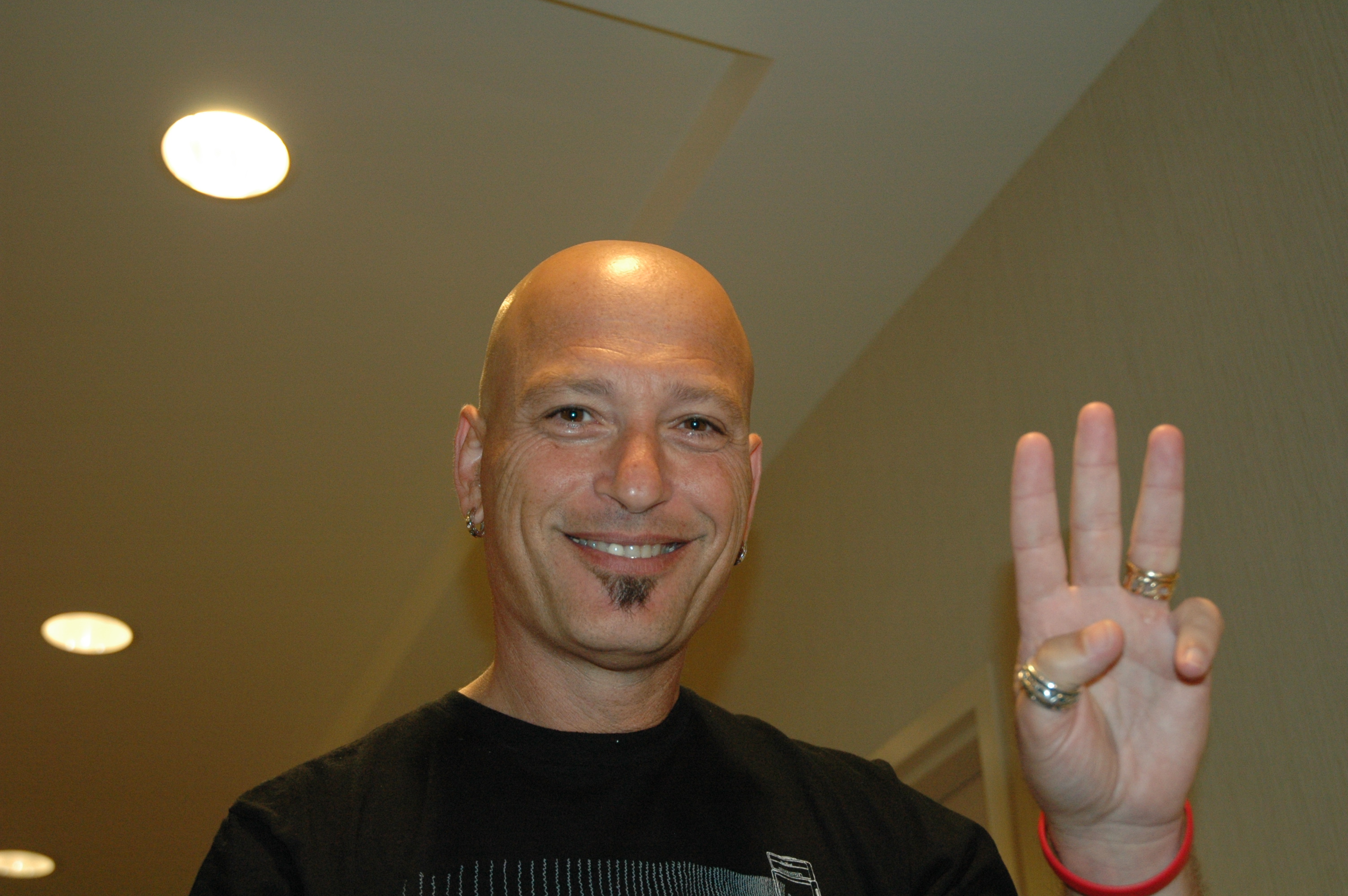In this image, Howie Mandel, the well-known comedian and TV host, is the focal point. The photo is taken from a low angle, capturing Mandel from below and including the room's ceiling and overhead lights in the background. Howie Mandel, a white man likely in his late 50s or early 60s, is instantly recognizable with his bald head, a small soul patch, and earrings. He is dressed casually in a black shirt, adorned with a couple of rings on his fingers and a red wristband. Striking a playful pose, Mandel is holding up three fingers in a gesture reminiscent of a peace sign, but with an added finger. His smile adds to the casual, friendly vibe of the picture.